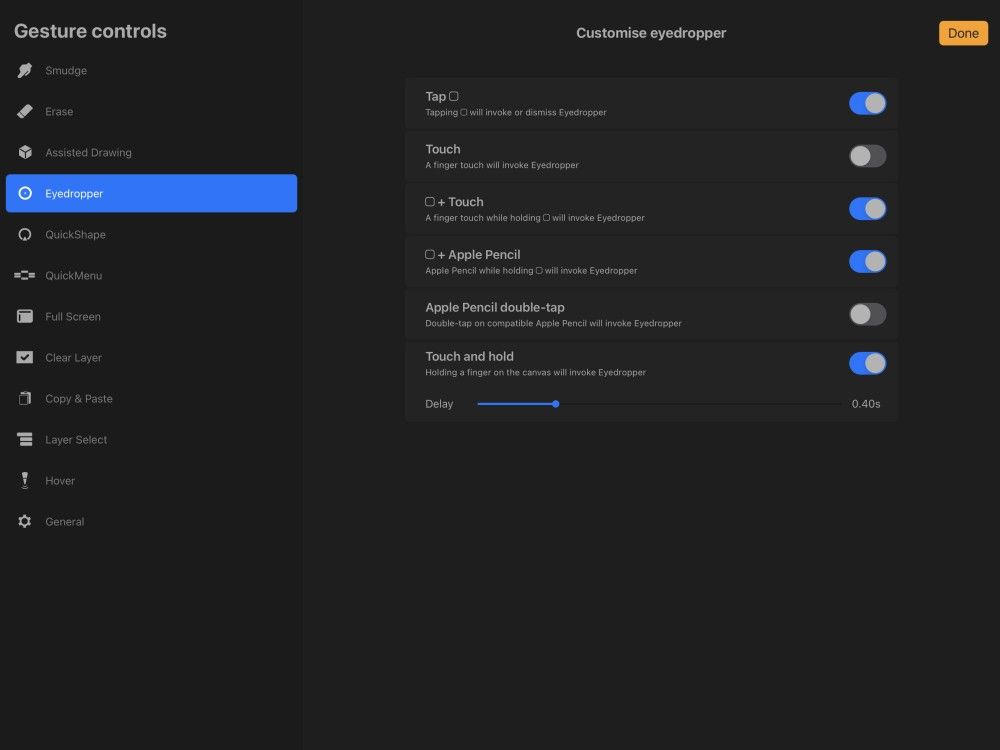The image depicts a control panel specifically designed for gesture controls within a graphics program. In the upper left corner, the words "Gesture Controls" are prominently displayed. This panel includes a comprehensive list of tools, each represented by an icon, which are: Smudge, Erase, Assistive Drawing, Eyedropper, Quick Shape, Quick Menu, Full Screen, Clear Layer, Copy and Paste, Layer Select, Hover, and General.

On the right side of the panel, there is a section titled "Customize Eyedropper" with an orange button labeled "Done" located in the upper right corner. Below this section are seven rectangular tabs, each equipped with sliders that can be toggled on or off. When the slider is on, it is moved to the right and turns blue; when off, it is moved to the left and turns gray.

The customization options for the eyedropper tool include:
1. Tap: "Tapping will invoke or dismiss eyedropper" is currently set to on.
2. Touch: "A finger touch will invoke eyedropper" is set to off.
3. A key plus touch: "A finger touch while holding a specific key will invoke eyedropper" is on.
4. Another key plus Apple Pencil: "Using the Apple Pencil while holding this button will invoke eyedropper" is on.
5. Apple Pencil Double Tap: "Double tapping a compatible Apple Pencil will invoke eyedropper" is off.
6. Touch and Hold: "Holding a finger on the canvas will invoke eyedropper" is on, with a delay of 0.40 seconds controlled via an adjustable slider.

The overall design of the panel features various shades of dark gray, providing a visually consistent and professional look conducive to creative work.